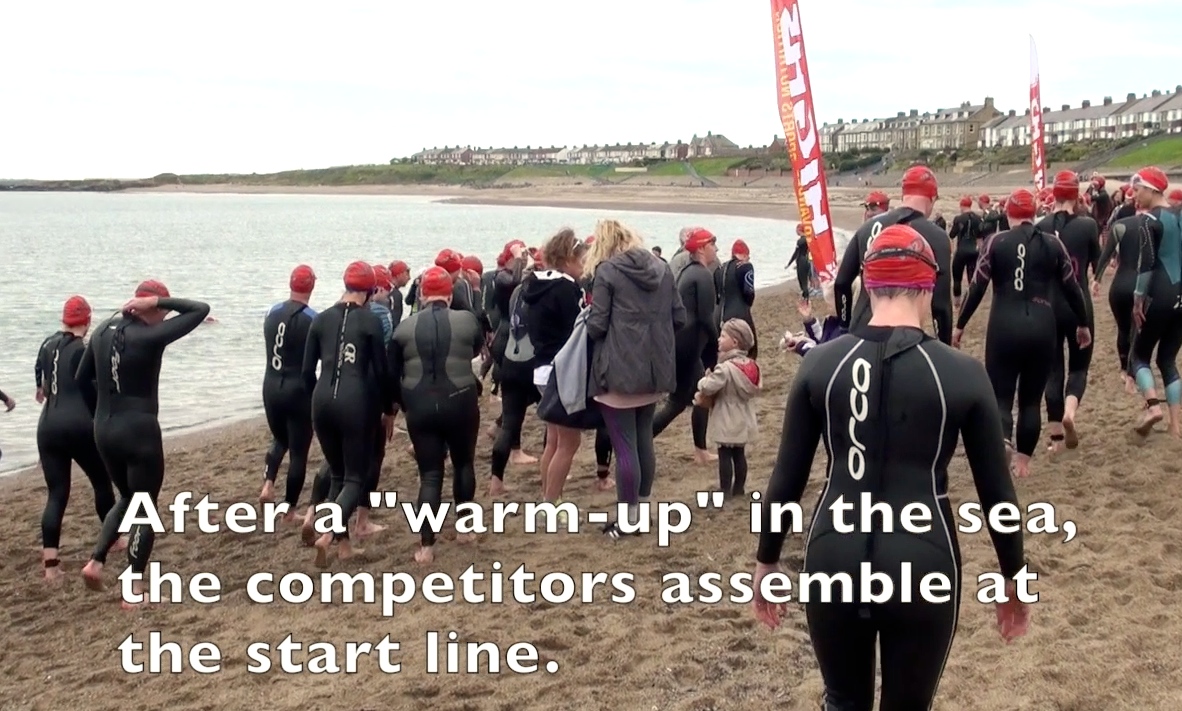In the foreground of this detailed photograph, a group of women clad in skin-tight black swimsuits, each adorned with orange-colored shower caps, strides across soft sand. The prominent figure on the right bears a black strap with the letters "O-R-C-A" running vertically, and her swimsuit features white lines tracing her silhouette. She's looking down with her hands resting by her hips. The soft sand beach they traverse curves around to the left, meeting light green, slightly rippling water. In the distant background, tall white and brown buildings, possibly condos or hotels, rise two to three stories high. Centrally positioned are two women not in swimsuits: one in a grey coat with purple pants and a black suit with shorts, the other with blonde hair, accompanied by a child dressed in a light cream jacket and brown pants. The white caption at the bottom reads, "After a warm-up in the sea, the competitors assemble at the start line," suggesting a race or competition. Scattered orange signs likely indicate the start line. The overall setting combines beachfront serenity with the spirited anticipation of the event.